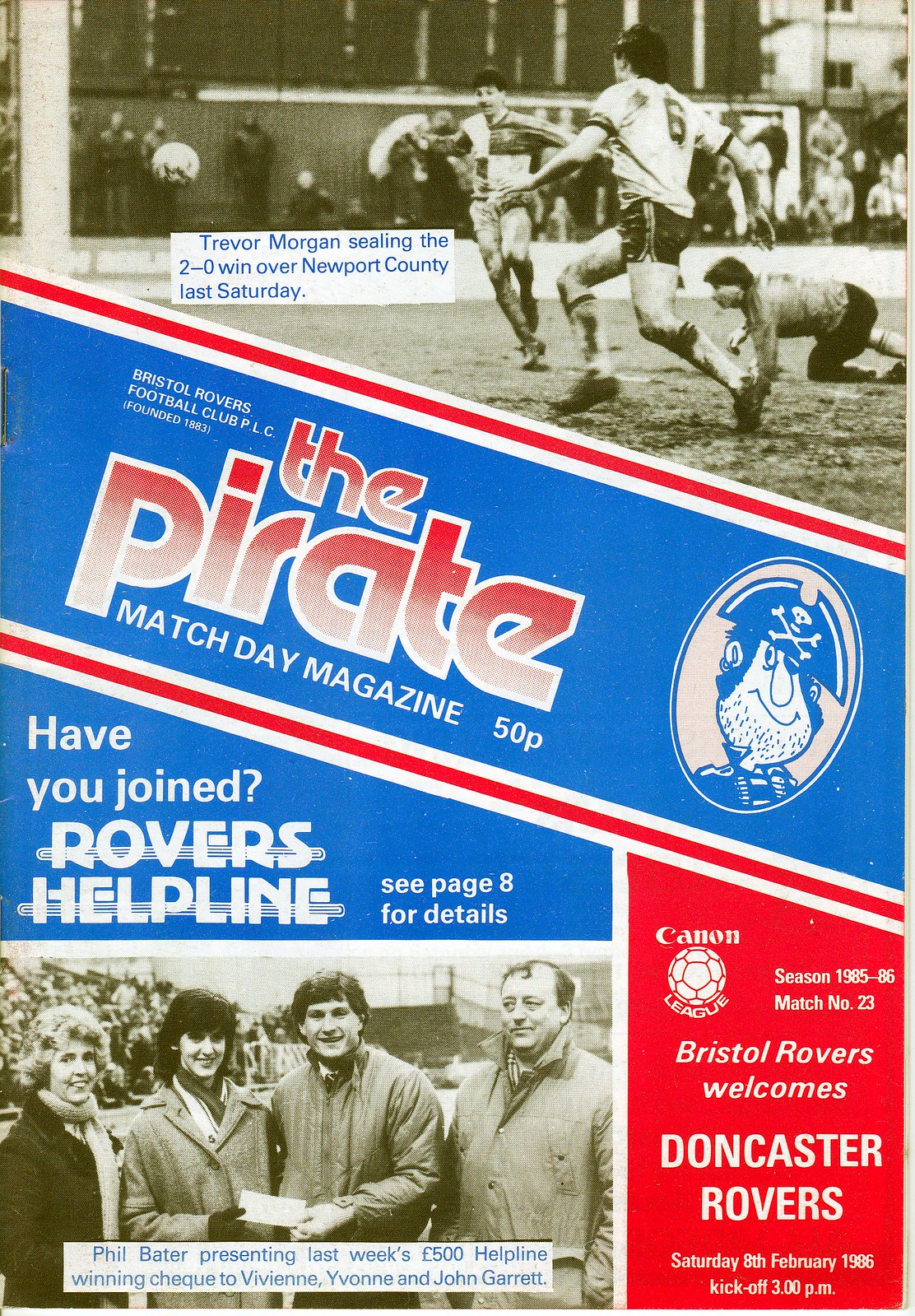This is the cover of an old game program for a soccer match. At the top, there is a black and white photo with a slight brownish tint, showing three men in t-shirts and shorts engaging in a rugby game amid muddy conditions. The player on the right appears to have fallen. The accompanying caption reads, "Trevor Morgan sealing the 2-0 win over Newport County last Saturday."

Diagonally across the middle of the cover, there is a blue banner with red and white borders, displaying the title "The Pirate" in a gradient of red to white letters. Below the banner, it says, "Bristol Rovers Football Club, PLC, Founded 1883," and "Match Day Magazine, 50p."

On the right, there is an oval white circle containing a cartoon drawing of a pirate from the shoulders up. Below this, text reads, "Have you joined Rovers Helpline? See page 8 for details."

Toward the bottom of the cover, there is another black and white photo of four individuals wearing outdoor pea coats, captioned, "Phil Bader presenting last week's £500 helpline winning cheque to Vivian, Yvonne, and John Garrett."

On the lower right, there is a red section with tiny letters that reads, "Canon League" with a soccer ball icon between the words, alongside "Season 1985 to 86, Match Number 23, Bristol Rovers welcomes Doncaster Rovers, Saturday, 8th February 1986, Kickoff 3:00 PM."